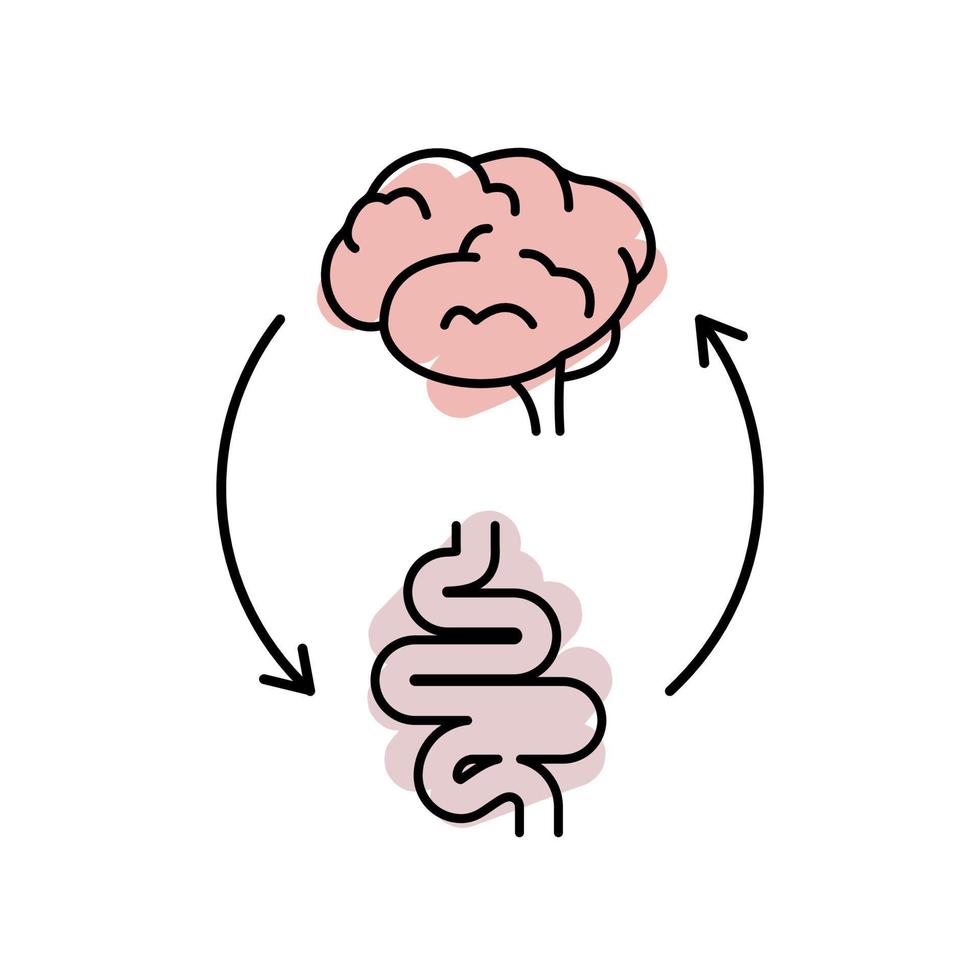This detailed digital line drawing on a white background illustrates the connection between the brain and the digestive system. At the top, a brain is depicted with black outlines and a pinkish hue, focusing on the right hemisphere and including the brain stem. Below, the digestive tract is shown, beginning with the esophagus curving into an 'S' shape leading to the stomach, and continuing into the intestines, colored in a lighter, almost purplish pink. Two black arrows are drawn to emphasize the bidirectional communication between the brain and the digestive tract; one arrow points down from the brain to the intestines, while another points up from the intestines back to the brain. The layout somewhat forms a circular motion, indicating the influence of the brain on the digestive system and vice versa.